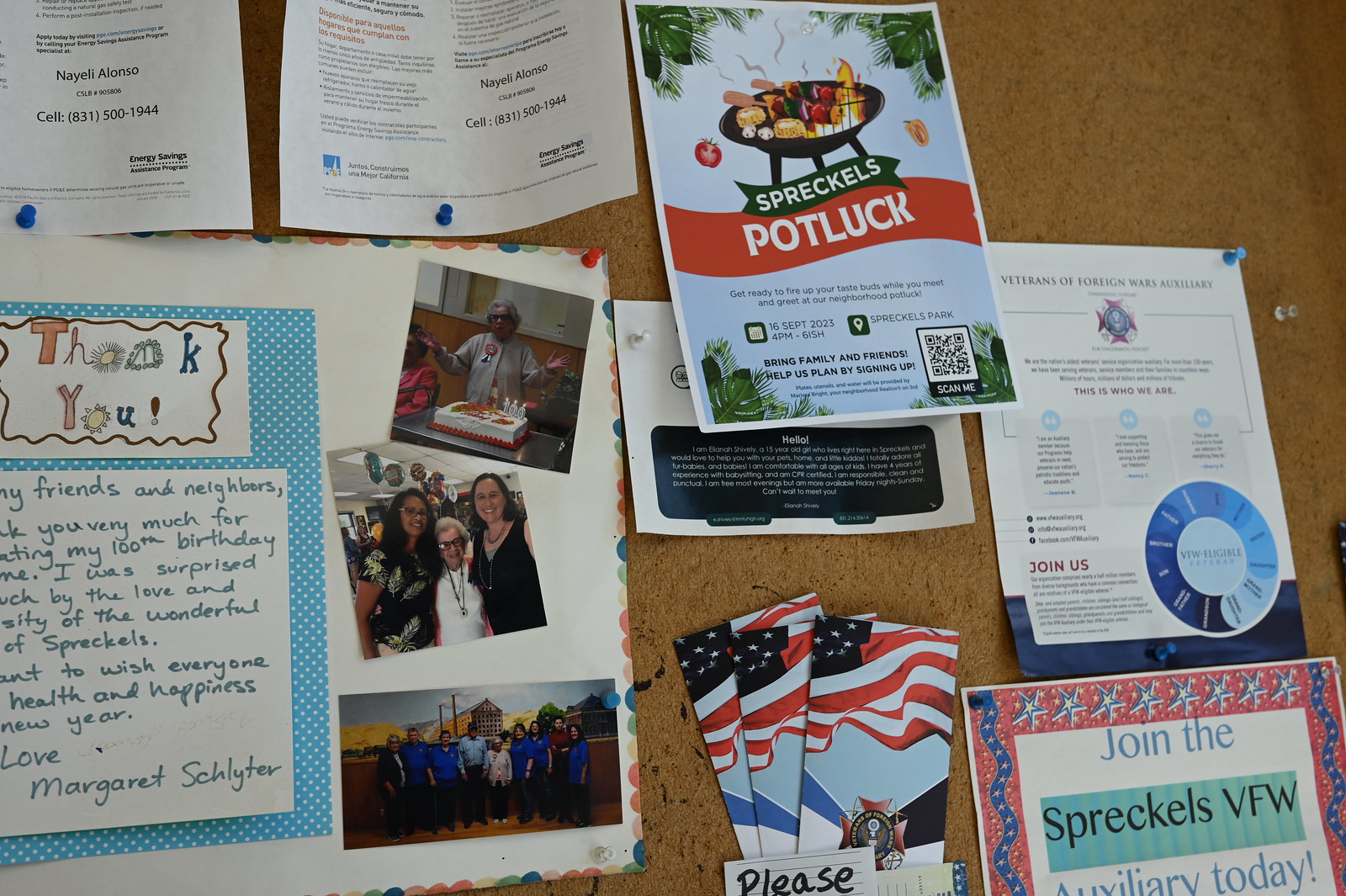This color close-up photo captures a bustling bulletin board at the VFW Hall in Spreckles. The cork board, a classic tannish hue, is adorned with a variety of flyers, pamphlets, and photos, all secured by pushpins in colors like dark blue, red, clear, and light blue. Prominently featured on the left-hand side is a heartfelt thank you note from Margaret Schleiter, surrounded by three photographs, expressing her gratitude to friends and neighbors for making her 100th birthday celebration memorable. Margaret also wishes everyone health and happiness in the new year. Below this, on the bottom right, is a flyer encouraging people to "Join the Spreckles VFW Auxiliary Today." Centered on the board is a vibrant flyer for the Spreckles Potluck, complete with a colorful image of a grill and cooking meat, inviting the community to bring family and friends and sign up via a QR code labeled "scan me." Additionally, several white paper flyers with small print and brochures featuring the American flag add to the patriotic theme, while another flyer includes a circle graph promoting the Veterans of Foreign Wars Auxiliary. The overall scene is a testament to the active and communal spirit of the Spreckles community.